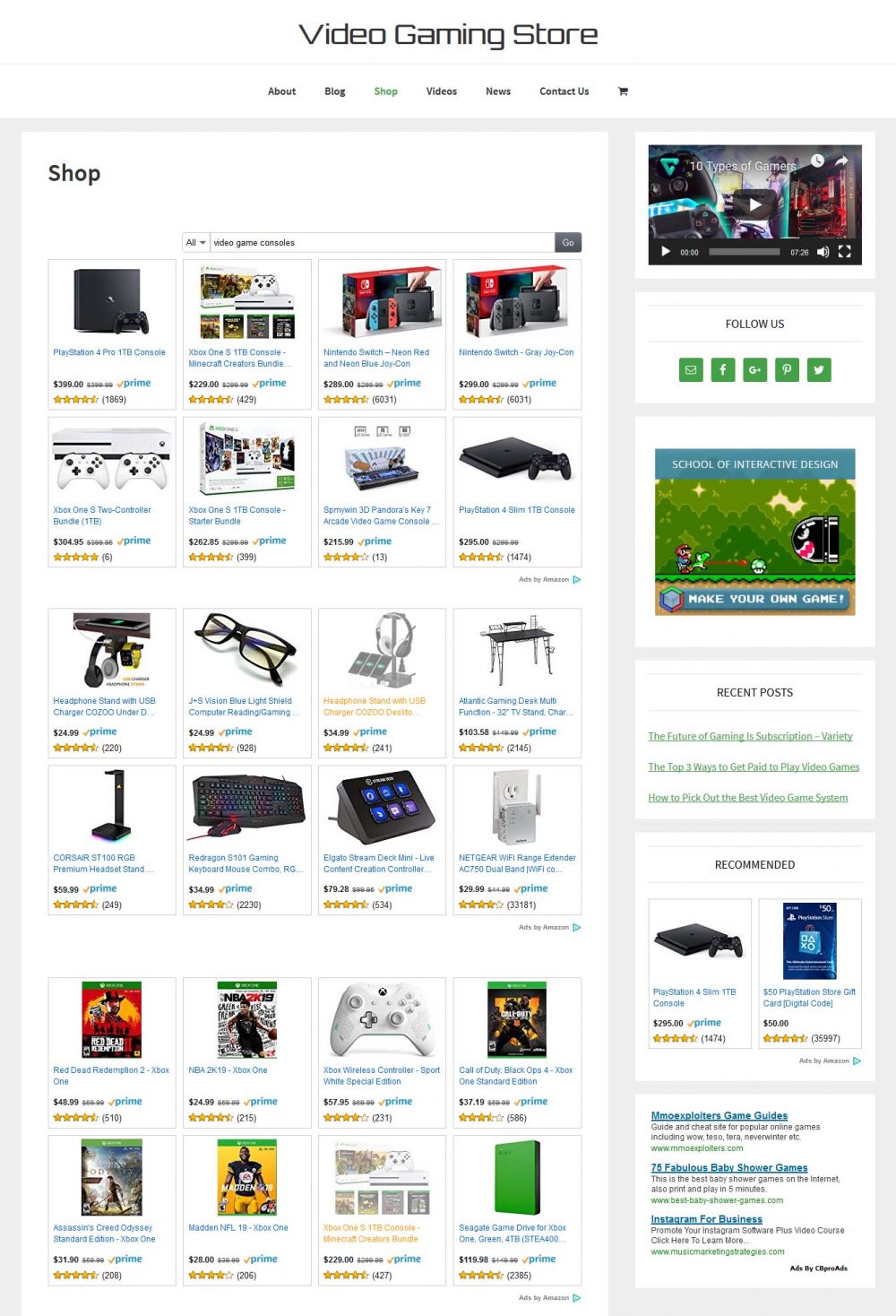The image captures a vibrant display in a Video Gaming Store, effectively laid out to guide enthusiasts through various products available for purchase. At the top of the image, "Video Gaming Store" is prominently displayed in bold, black text. 

To the left side, set within a long rectangle, the word "Shop" is also rendered in black text, inviting customers deeper into the array of offerings.

The store is systematically organized into different rows showcasing an array of gaming products. In the first row, a boxed Nintendo Switch package is highlighted, featuring the console along with its distinctive red and blue Joy-Con controllers.

Moving to the second row, sleek white controllers with contrasting black buttons are displayed, with a PlayStation console visible on the far right of the same shelf.

The third row deviates slightly from gaming consoles and controllers, presenting a stylish pair of black eyeglasses.

Next, the fourth row reverts to technology with the Amazon Show prominently showcased, boasting its smart display capabilities.

Beneath this, a collection of Xbox video games is strategically placed. These games are easily identifiable by the green banner at the top, giving away their Xbox association. One of the games, presumably a sports title, is adjacent to a crisp white Xbox controller.

Finally, on the bottom row, numerous games are presented, with one particularly drawing attention—a football game featuring a player in yellow pants is marked by a green header. To the right of this, a variety of other gaming options are available, culminating in a captivating centerpiece: a screenshot from a Mario game, vividly depicting a large black Bullet Bill with menacing eyes and a wide mouth bearing down on Mario.

The well-organized layout and diverse range of products cater to every gaming aficionado's needs, making for a visually appealing and comprehensive shopping experience.